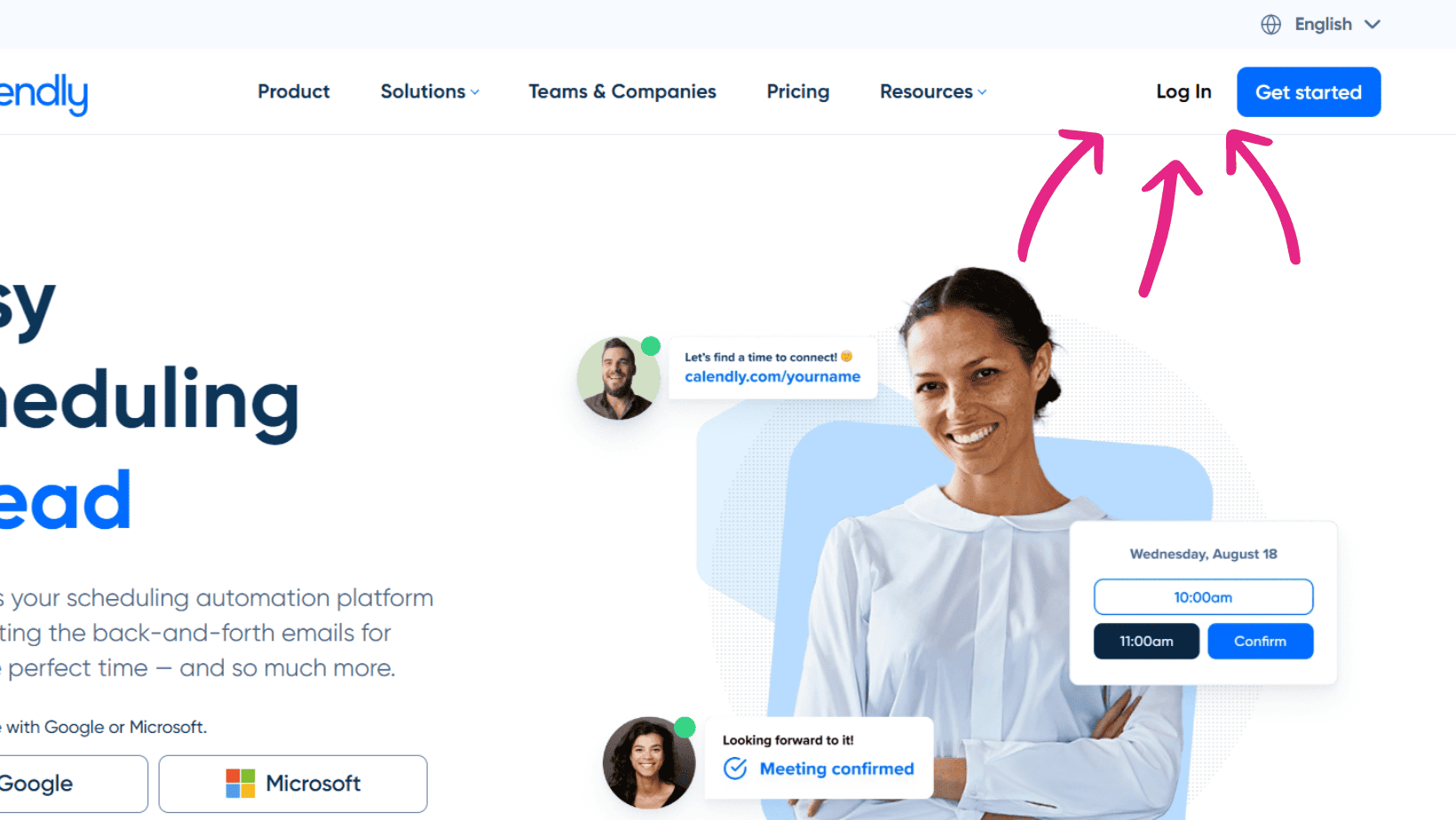The image displays a partially cropped webpage of a meeting scheduling tool, presumably named "Calendly", as suggested by the visible letters "E-N-D-L-Y" in the upper left corner. In the top section of the webpage, a navigational menu is present with headings such as "Product", "Solutions", "Teams and Companies", "Pricing", and "Resources." Some of these headings appear to have dropdown menus, indicated by small carets. Additionally, there is a "Log In" option highlighted by three hand-sketched pink arrows, and a blue "Get Started" button.

At the center of the webpage is a prominent section featuring a black woman in two different photos. In one image, she is wearing a white blouse with no collar and a tight neckline. To her left are two circular avatar icons with headshots inside. One of the avatars depicts a bearded man with a green dot next to his image, suggesting he is online. He has a speech bubble next to him that says, "Let's find a time to connect," followed by a link to "calendly.com/yourname". 

The lower part of the image shows what appears to be the same woman, but this time with her hair down and wearing a black top. A matching dialog box indicates that a meeting has been confirmed with the text, "Looking forward to it!" along with details specifying the meeting date and time as "Wednesday, August 18" at "10 a.m." and a "Confirm" button right next to it.

Overall, the composition of the webpage is clean and interactive, designed to facilitate the scheduling of meetings in a user-friendly manner.